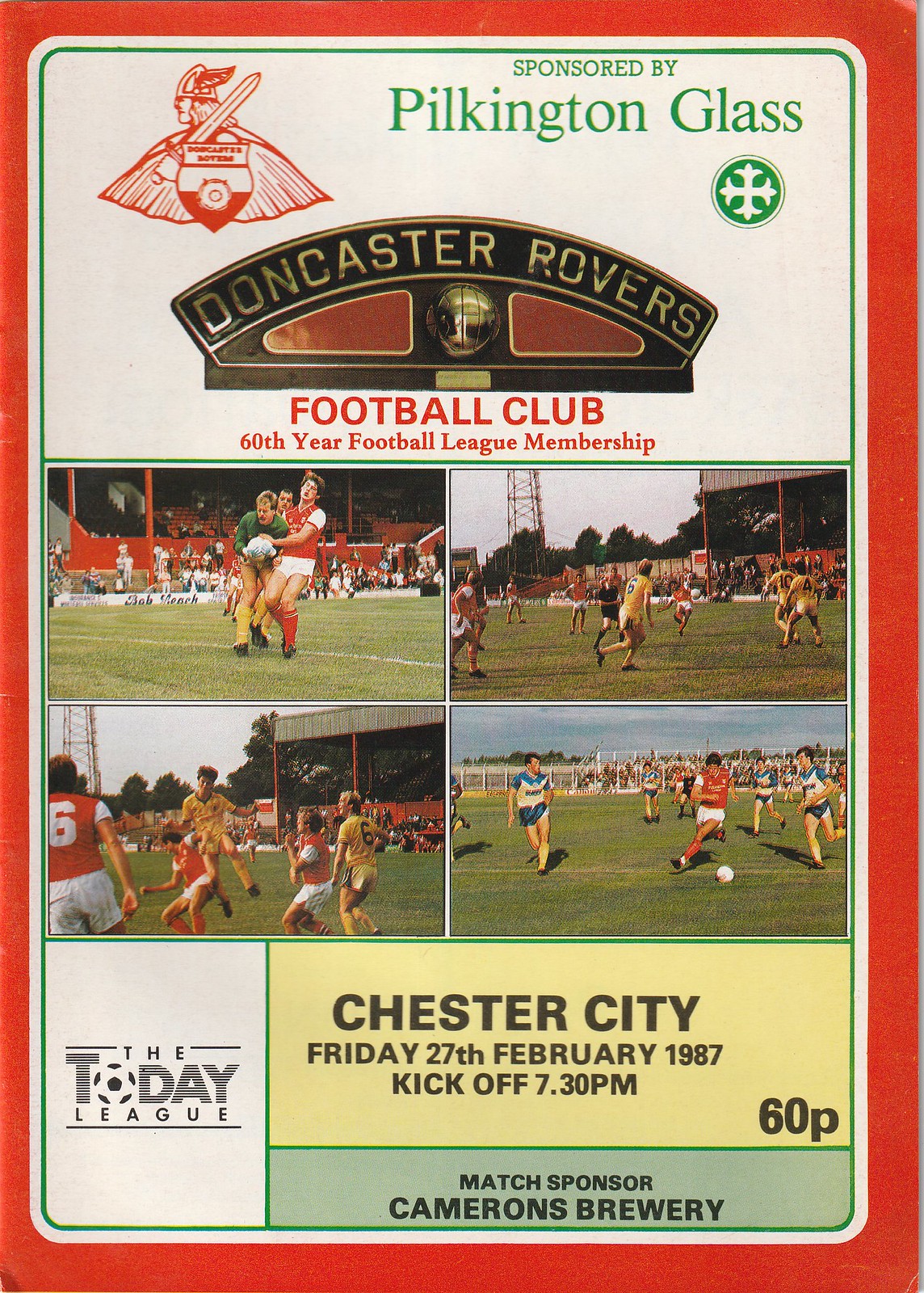The rectangular image, which appears to be the cover of a sports program or small magazine, features a vibrant red outline and is divided into multiple boxes. At the top, a large green-outlined box houses an emblem of a warrior holding a sword and shield with unreadable red text on a white background. Next to the emblem, “Sponsored by Pilkington Glass” is prominently written in green, accompanied by a small business symbol. Below this, a black background showcases the name “Doncaster Rovers” in gold lettering, flanked by a gold soccer ball, with the phrase “Football Club 60th Year Football League Membership” written in red below it.

The lower half of the cover is organized into four smaller boxes containing mid-game soccer action shots. These images depict players predominantly in red uniforms engaging in various plays. At the bottom left, on a white background with black print, it reads “the Today League” with the O replaced by a soccer ball. Adjacent to these boxes, a larger yellow-background box announces “Chester City, Friday, 27th February 1987, kickoff 7:30 p.m., 60p.” Beneath this, in a smaller green-background box, the match sponsor “Cameron’s Brewery” is noted.